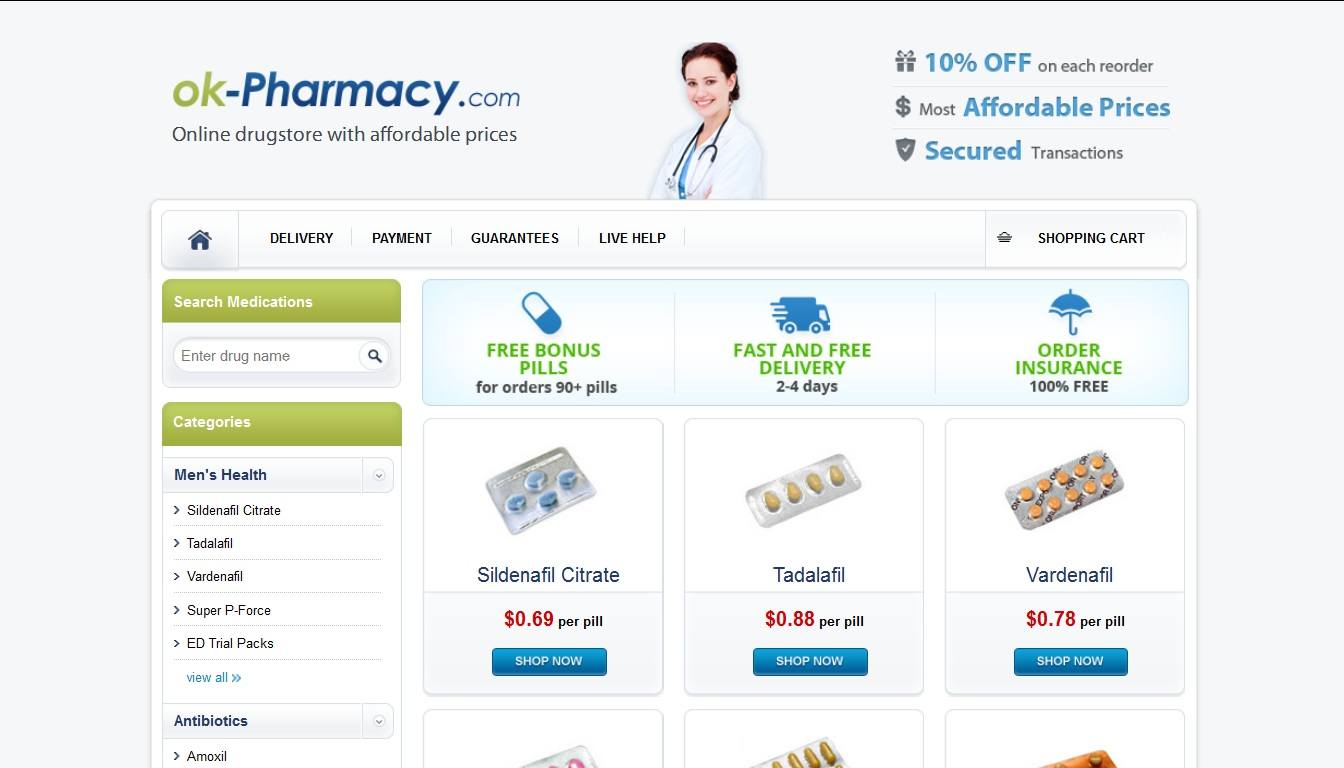The image depicts a webpage for OKPharmacy.com, an online drugstore boasting affordable prices. The webpage features a clean, white background accented with green and dark blue elements. In the top left corner, the website's name is prominently displayed, with "OK" in green and "pharmacy.com" in dark blue. Below, a tagline reads "Online drugstore with affordable prices."

At the center of the page stands a smiling female doctor with dark brown hair tied back, wearing a white coat and a stethoscope around her neck. Her arms are folded across her midsection, exuding a welcoming demeanor.

To the doctor's right, there is a promotional text offering "10% off on each order," accompanied by a gift graphic and a gray money sign. The phrase "most affordable prices" is highlighted in blue. A blue shield icon signifies secured transactions, with the text in gray.

Navigation buttons are located at the top of the page, including options for Home, Delivery, Payment, Guarantees, and Live Help. Additionally, there is a shopping cart icon and a search bar for medications, styled in green with "categories" also listed in green. A promotional banner at the bottom announces "Free bonus pills for every 90-plus orders," illustrated with a graphic of a pill.

Overall, the webpage exudes a trustworthy and professional aesthetic, aiming to attract customers with its affordable prices and secured services.